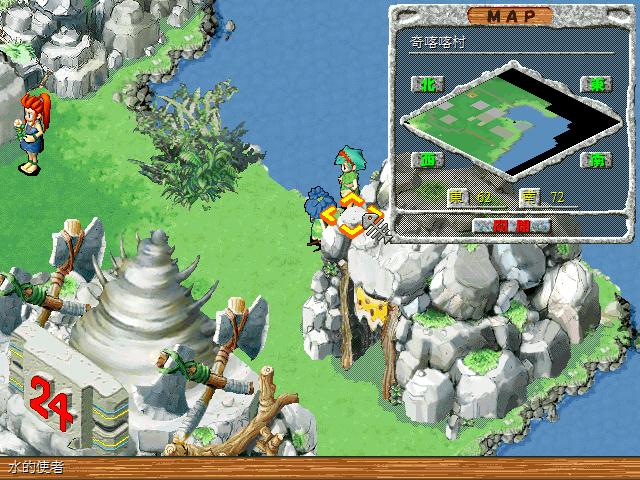The image resembles a video game screen. In the upper right corner, there is a mini-map, bordered by a brown margin along the bottom, which features characters from an unfamiliar language. The mini-map displays a large green area representing land and a smaller blue area depicting water, bordered by black. Adjacent to the mini-map, various small icons in gray, yellow, and green can be seen.

Dominating the screen is a larger, detailed depiction that mirrors the mini-map's layout, showing the extensive green land and the smaller blue water area. The black-shaded region from the mini-map is not visible in this cropped image. Upon closer inspection, the scene reveals stone-built huts with wooden door frames, adding a rustic feel. Prominently featured is a woman or girl with red hair, adorned in a blue dress, and holding a pink flower, adding a vibrant human element to the scene.